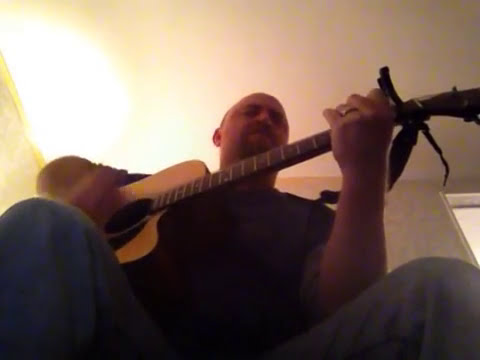In the image, an adult male is playing an acoustic guitar while seated, with the photograph taken from a low angle, looking up towards him. This unique perspective captures the man almost filling the entire frame, emphasizing the underside of his chin and the bottom of the guitar. He is dressed in a black shirt and blue jeans, with his legs spread apart, revealing his knees. His left hand is positioned on the chords, adorned with a wedding ring, while his right hand is in motion, strumming the strings, creating a motion blur over the guitar's sound hole. The man is bald with a closely cropped mustache and beard, and his eyes are closed, suggesting a deep connection with the music. The background reveals a white ceiling illuminated by a bright light over his right shoulder, casting a significant glow. To the right edge of the frame, a doorway is just barely visible, while a window on the wall is discernible to his left. The detailed textures of the wooden guitar add an earthy tone to the scene, merging seamlessly with the ambient light and subtle room details.